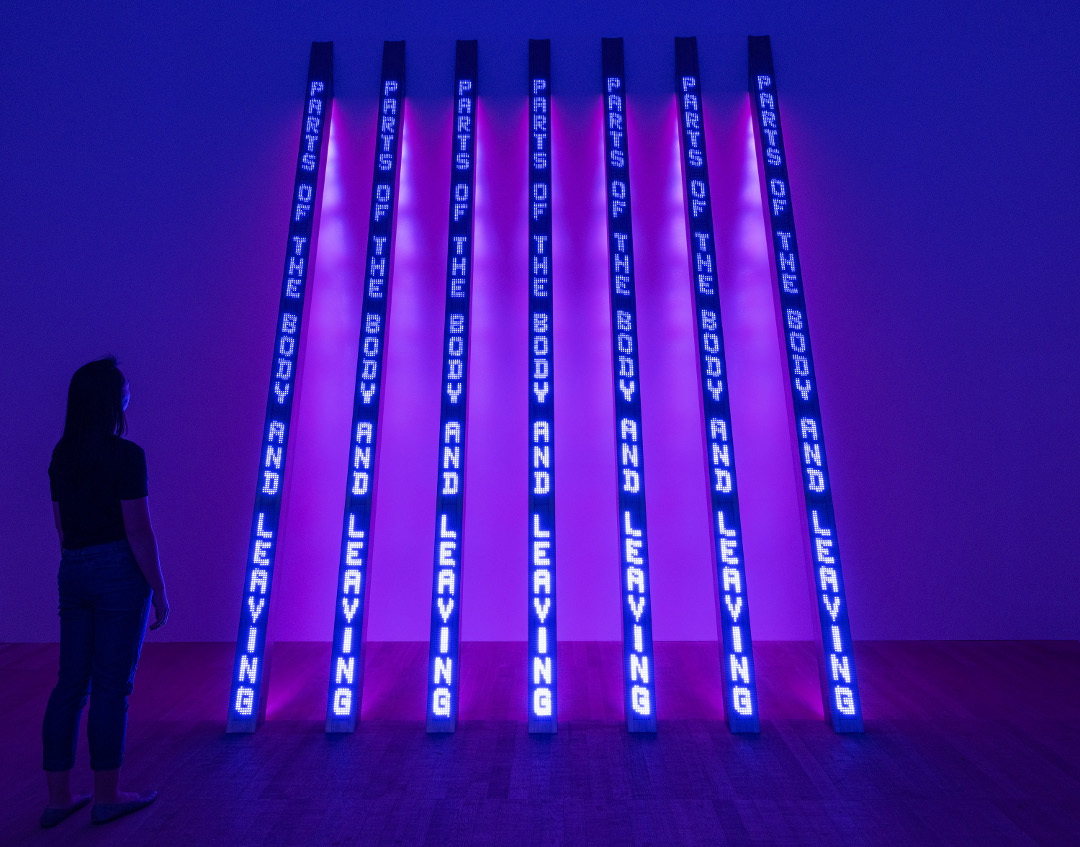The image depicts a woman standing at the bottom left against a darkened backdrop. She has shoulder-length dark hair, is wearing a short-sleeved black shirt, lighter-colored jeans, and flat slip-on shoes. The wooden floor beneath her is composed of vertical wooden panels.

In front of her and leaning against a wall are seven tall black rectangular objects, each illuminated by white text in blue neon lights that read, “parts of the body and leaving.” These objects, illuminated from behind by a purple light, cast a purplish glow on the wall. The text on the banners is vertically oriented, running from top to bottom. The overall scene is dimly lit, with the primary sources of light being the blue-front LEDs and the purple backlighting. The objects appear to be approximately two and a half times the height of the woman.